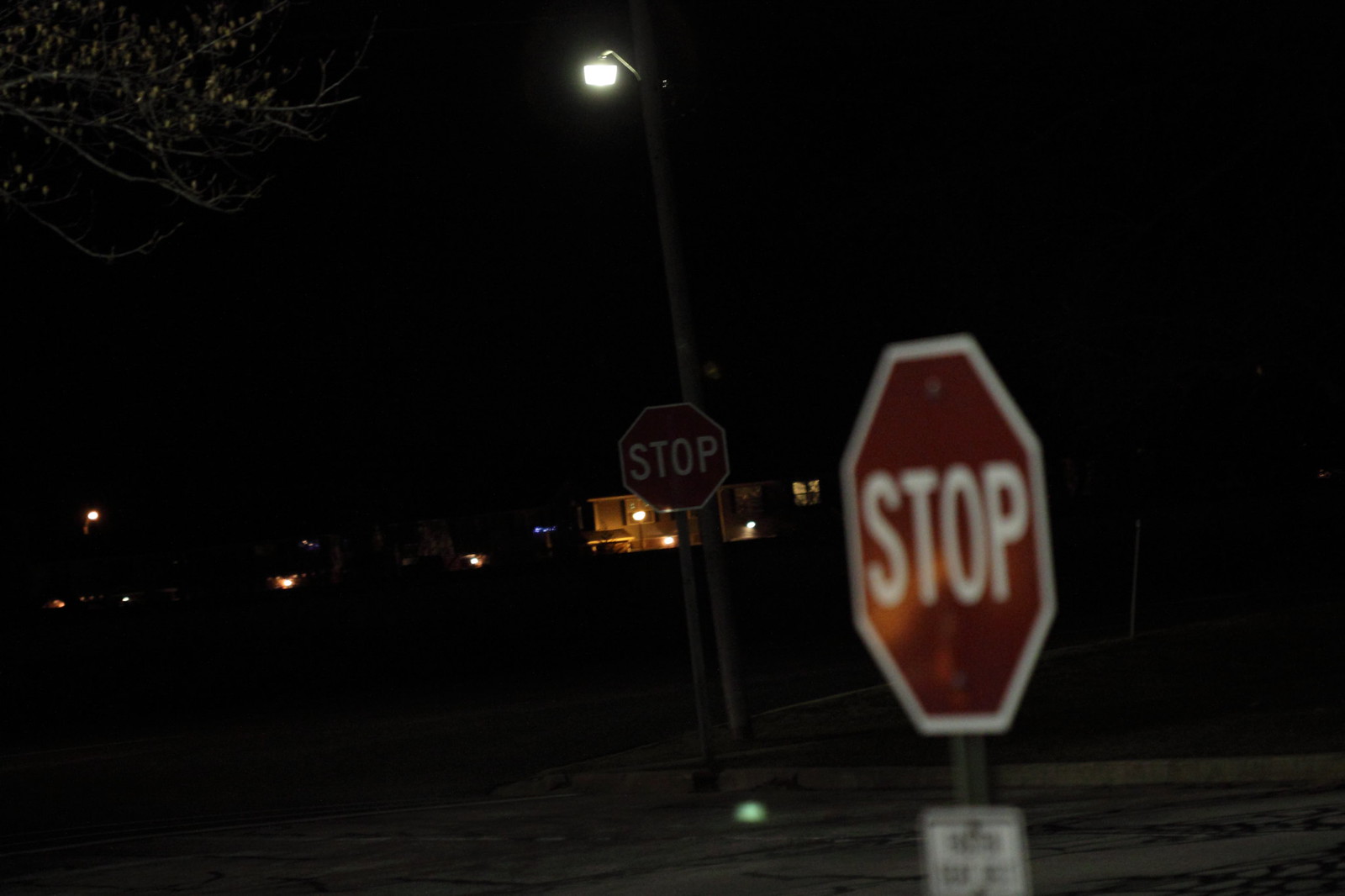This nighttime photograph captures a dark, dimly lit street intersection. Dominating the right-of-center foreground is a slightly out-of-focus, red stop sign reflecting light. Beneath this stop sign is an unreadable white notification sign, equally blurred. Further back near the center of the image is another stop sign, smaller in appearance due to its distance, and also difficult to see amidst the shadows. The backdrop reveals faint lights, highlighting what seems to be a residential house with some lit windows. At the top of the image, a bright street light bathes the area in a stark glow, and the wet street below reflects its illumination. The upper left corner showcases the silhouette of tree branches. Scattered in the middle distance are additional, indistinct lights contributing to the scene's urban nightscape.